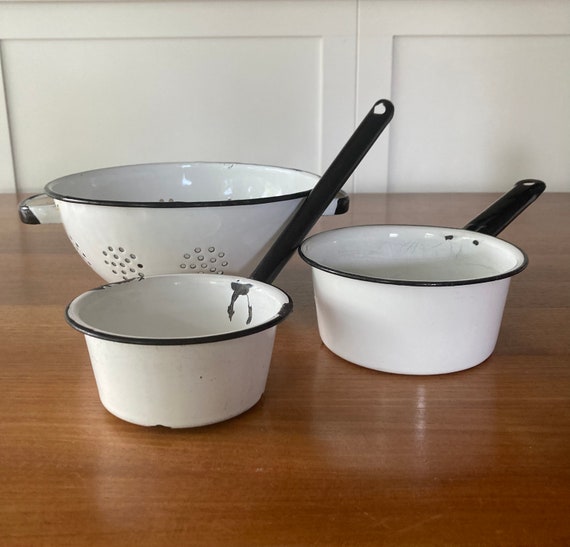The image captures a rustic kitchen scene featuring three pieces of well-worn white enamel cookware, detailed with black handles and rims, resting on a polished brown wooden table. Two are saucepans, with long black handles ending in holes for hanging, showing signs of age with chips and scuffs in the porcelain. Positioned behind the smaller saucepan is a matching white colander, identifiable by its numerous straining holes and dual side handles in black and white enamel. In the background, two white wooden cabinetry panels provide a clean, simple backdrop to the vintage cookware ensemble.